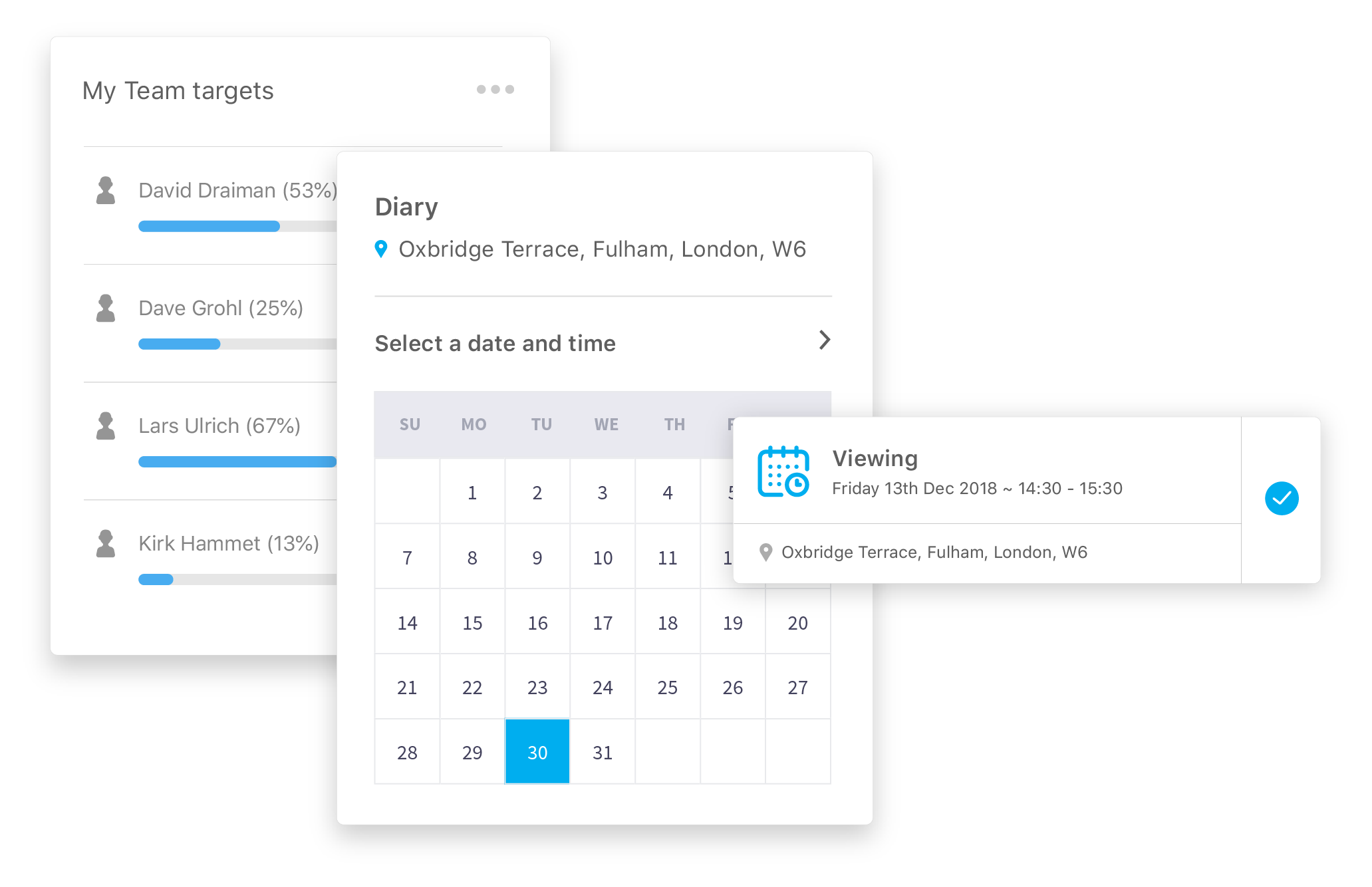The image depicts a detailed interface for team targets and a calendar event. At the top, a white rectangle with gray lettering reads "My Team Targets," accompanied by a light gray three-dot dropdown menu icon. Enclosed by a light gray border, the interface lists team members and their target completion percentages: David Draymond (53%) with a half blue, half gray progress bar, Dave Grohl (25%), Lars Ulrich (67%), and Kirk Hammett (13%).

Additionally, a slightly overlapping square or rectangle labeled "Diary" in bold lettering features a light blue map pin icon with text reading "Oxbridge Terrace, Fulham, London, W6." Further down, a dark gray text heading, "Selected Date and Time," appears beside a right-pointing arrow. Below this heading, a calendar displays days from 1 to 31, with the 30th highlighted in blue and featuring the number in white text.

An overlay displays a long rectangle labeled "Viewing" next to a calendar and clock icon. This section specifies "Friday, 13 December 2018" and the time range "14:30 - 15:30." To the right of this overlay is a blue check mark symbol, commonly associated with verification.